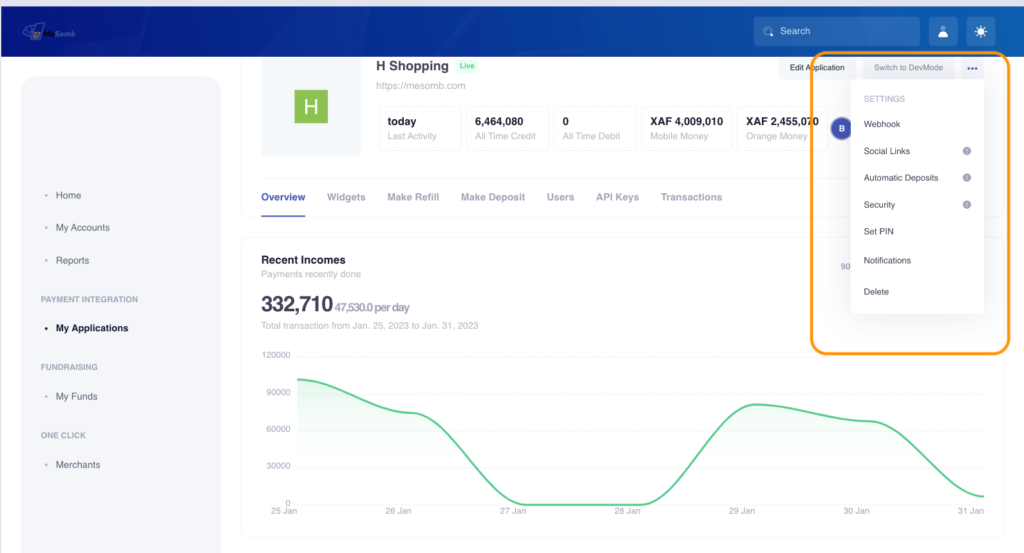This image depicts a detailed view of a website interface related to a financial management system, likely for an e-commerce platform named H-Shopping.

At the top of the webpage, there is a blue navigation bar that includes a search function, a profile picture, and a small circular sun-like icon. Alongside, it features assorted text elements: the company's name "H-Shopping" in prominent lettering, the word "Live" in green text, the domain "Meesom.com," and a note indicating that "the last activity was today."

Financial statistics are prominently displayed, highlighting an "All-time credit" of $6,464.80 and an "All-time debit" of zero. Subsections show specific balances for "mobile money XAF" at $4,009 and "orange money" at $2,455.70.

Functional buttons labeled "Edit Application" and "Switch to Dev Mode" appear, surrounded by an orange square, likely to draw user attention for interaction.

The settings menu presents various configuration options such as webhook, social links, automatic deposits, security, setting a pin, notifications, and a delete option.

The page also contains a section dedicated to "Recent Income," showcasing a significant amount of $332,710. Complementing this report is a green-colored graph charting "Total transactions from January 25th, 2023, to January 31st, 2023." The graph provides a visual representation of transaction activities ranging from 9,000 to zero over the specified dates.

The overall background of the page is predominantly white, emphasizing a clean and professional interface.